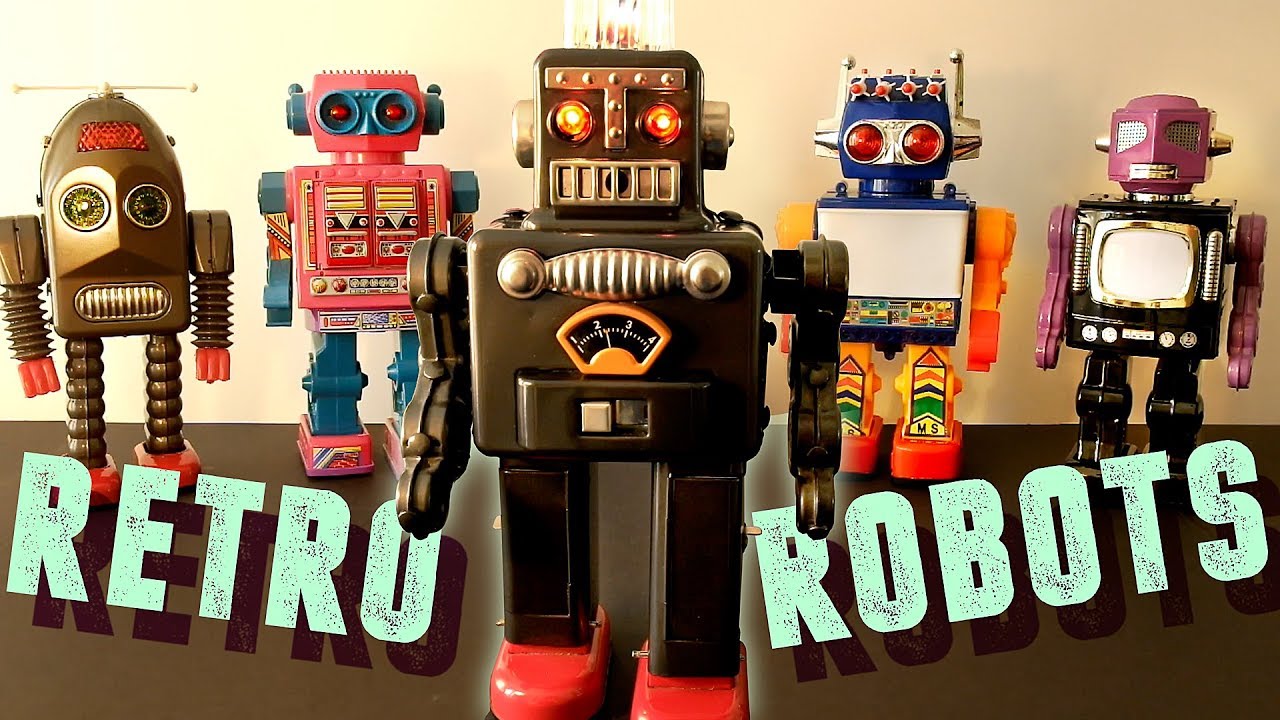This full-color, digitally enhanced photograph, horizontally rectangular and clearly staged with artificial indoor lighting, features five vintage-style toy robots aligned horizontally. Dominating the scene is a dark brown robot placed centrally, slightly ahead of the others. This central figure has a square head and body, complemented by a metallic, T-shaped gold detail on its face, red lights for eyes, and a grill-like mouth. A gauge with a needle pointing between 2 and 3 is centered on its torso, and it stands on red oval feet with one arm bent.

Directly to the left stands a whimsical brown and tan robot with a domed top, antenna-like rotors, circular eyes, and a grill for a mouth. Its red-capped, accordion-like arms and beaded legs give it a retro look.

To the right of the central robot is a futuristic robot with a rounded head featuring a blue background and glowing red eyes. It boasts a square body with a schematic and a white screen, paired with bright orange arms and legs.

Next in line is a compact robot characterized by pink and silver features, including metallic bolts and grated panels for eyes. A prominent TV-like screen occupies its chest, accompanied by knobs underneath.

The final toy robot on the far right has pink claws and brown legs with knee joints. It possesses pink arms and what appears to be a metallic TV screen on its belly.

The text "RETRO ROBOTS" is prominently displayed in bold blue capital letters at the bottom of the photograph, flanking the central robot, with "RETRO" on the left and "ROBOTS" on the right.